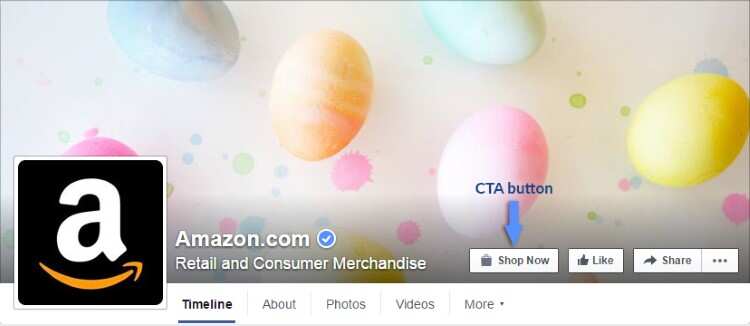This image appears to be a screenshot intended as an instructional guide. The background prominently features a photograph of decorated Easter eggs placed on a white sheet of paper, which is adorned with pastel-colored paint splotches that harmonize with the hues of the eggs. Superimposed on this image is an interface resembling a Facebook profile, distinguished by the Amazon logo featuring a black background, a white "A", and an orange arrow. 

To the right of the logo, the text reads "Amazon.com" followed by a verified checkmark and the classification "Retail and Consumer Merchandise". Adjacent to this, there are several interactive buttons: a "Shop Now" button indicated by a shopping bag icon, highlighted by a blue arrow and text labeled "CTA button", a "Like" button with a thumbs-up icon, a "Share" button with an arrow icon, and an ellipsis button for additional options.

Above these buttons, a navigation bar features a bolded and blue underlined "Timeline" option, indicating it is the selected view. It is flanked by lighter text options for "About," "Photos," "Videos," and a drop-down menu for "More".